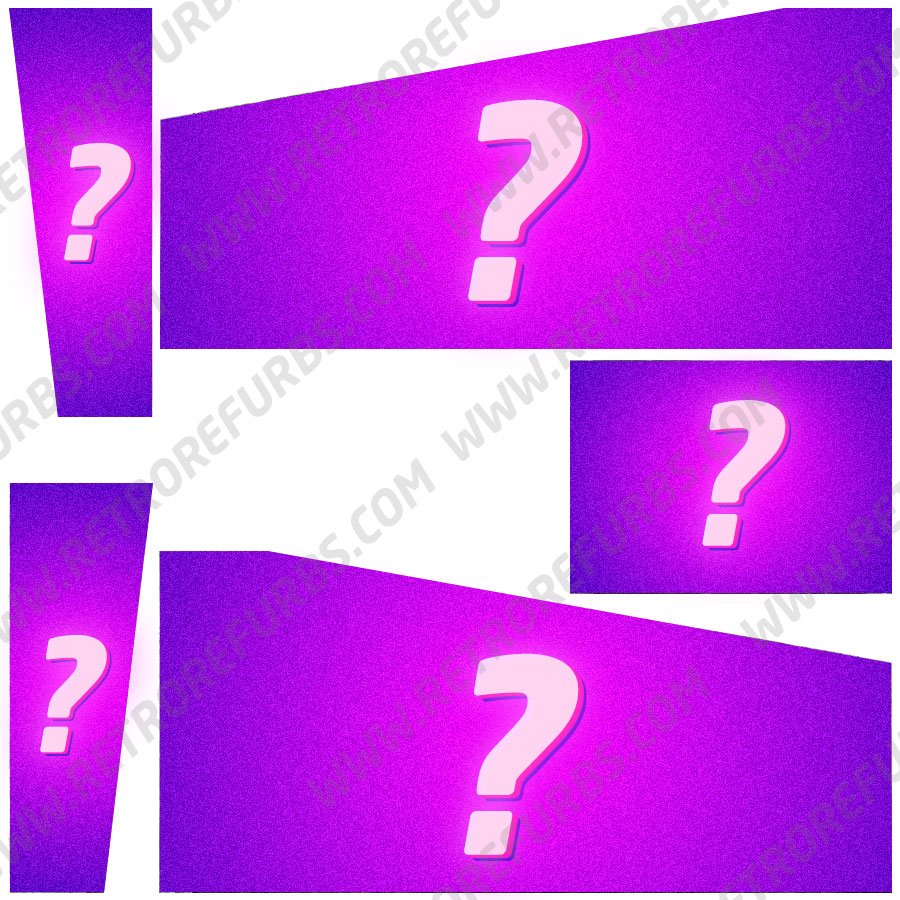The image is a perfectly square advertisement with a clean white background. Diagonal lines of gray text, difficult to read, span across with fragmented lettering, possibly spelling out "E-T-R-O-R-E-F-U-R" followed by "R-B". Six or seven diagonal lines extend from the left upwards to the right. Overlaying these lines are five shapes in shades of blue, purple, and pink, each distinct in color but blending where they meet. Each shape contains a white question mark centrally positioned. The top left and top right contain purple question boxes, while the bottom right and bottom left feature similar purple boxes. Additionally, two vertically oriented rectangles with wider tops are situated on the left, and one larger horizontal shape centrally placed, each enclosing a white question mark with blue and red outlines. The diagram's design ends with a perfect square in the middle also containing a white question mark, and the possible web address "www.retrofurbs.com" in the background.